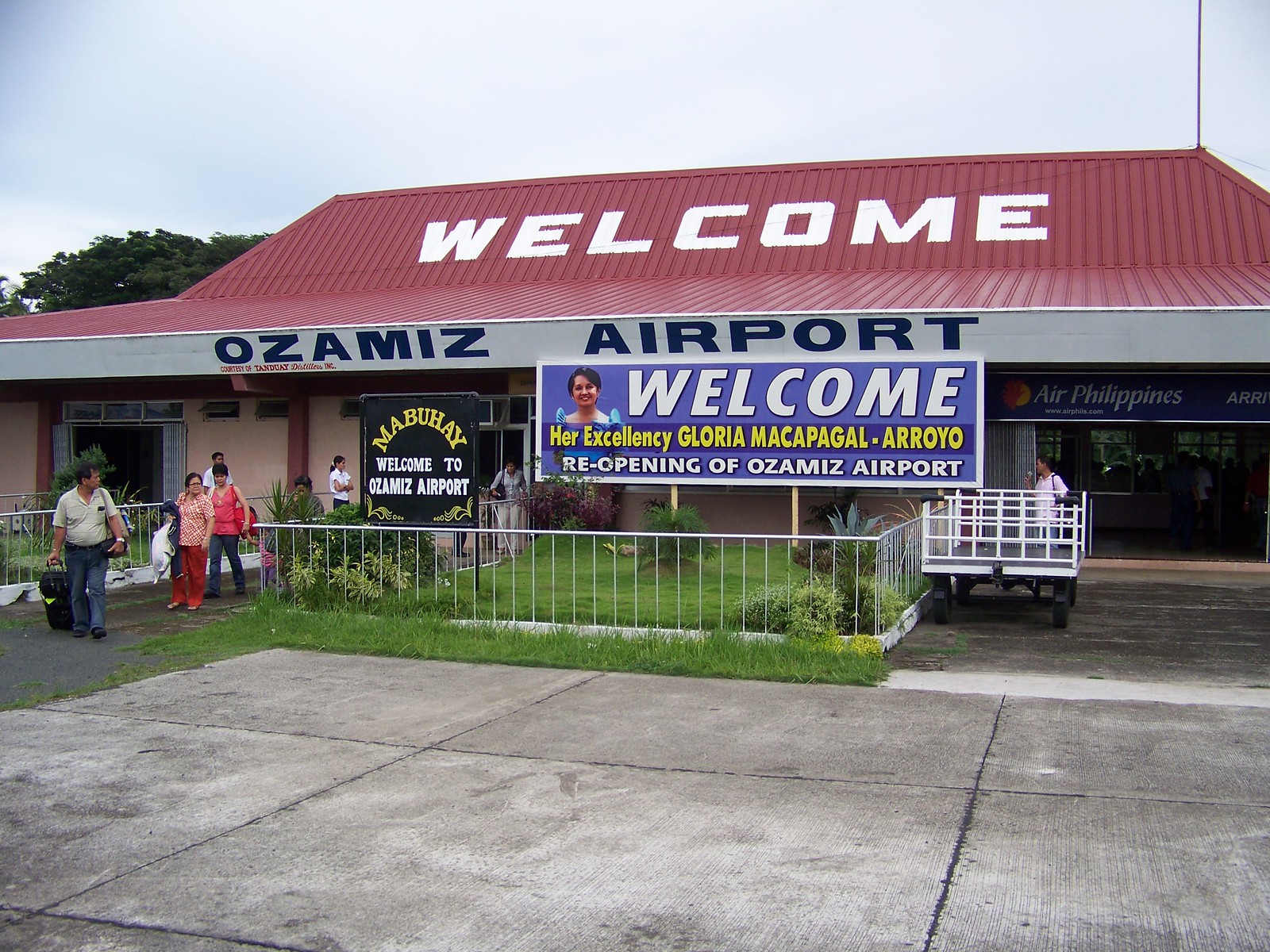This daytime photograph showcases the newly reopened Ozamis Airport, highlighted by bold white lettering on the red roof spelling out "Welcome" and "Ozamis Airport." A prominent black sign with white and yellow text, reading "Mabuhay, Welcome to Ozamis Airport," accentuates the entrance. Additionally, a large banner on the building welcomes Her Excellency Gloria Macapagal-Arroyo for the reopening ceremony. The scene captures a small courtyard with green grass and various plants, enclosed by a silver railing. Several people can be seen walking with their luggage across the gray concrete slabs in front of the airport, while a luggage carrying truck is visible on the right. Above, the partly cloudy sky adds to the vibrant daytime atmosphere, and a tree with lush green leaves stands in the distance.